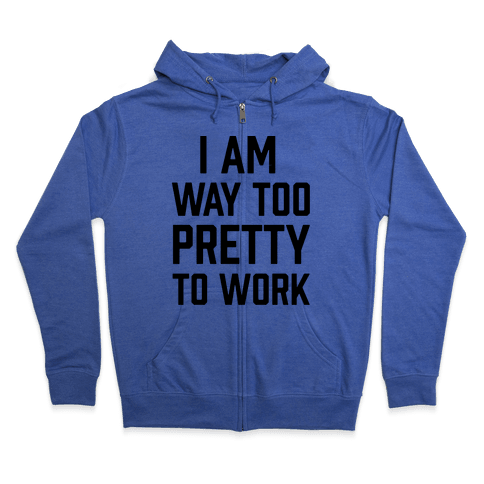This image showcases a bright blue zip-up hoodie, meticulously laid out flat against a pristine white background. The hoodie is fully zipped up, with its hood folded back and the sleeves positioned naturally downward. It features a pair of front pockets and a durable silver or gray zipper. The most striking detail of the hoodie is the bold, black, all-caps text emblazoned across the front, reading "I AM WAY TOO PRETTY TO WORK," with the word "PRETTY" slightly larger than the other words. The ends of the sleeves and the bottom hem of the hoodie have ribbing for flexibility, ensuring a snug fit. No additional elements or decorations are present, allowing the viewer to focus solely on the hoodie and its expressive statement.